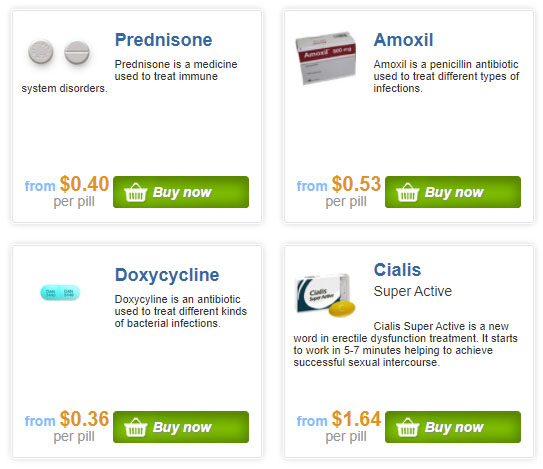The image depicts a section of a medication shopping site listing various prescription medicines. Each medication is detailed with its use, cost, and a purchase option. 

- **Prednisone**: Displayed as two circular tablets, this medication is used to treat immune system disorders. The price is listed at $0.40 per pill, and there is a prominent green "Buy Now" button.
  
- **Amoxil**: Shown in a generic box, this penicillin antibiotic is used to treat various infections. It is priced at $0.53 per pill.
  
- **Doxycycline**: Identified as an antibiotic for treating different kinds of bacterial infections, it is priced at $0.36 per pill.
  
- **Cialis Superactive**: Highlighted as a treatment for erectile dysfunction, this medication claims to start working within five to seven minutes to aid in achieving successful sexual intercourse. It is priced at $1.64 per pill.